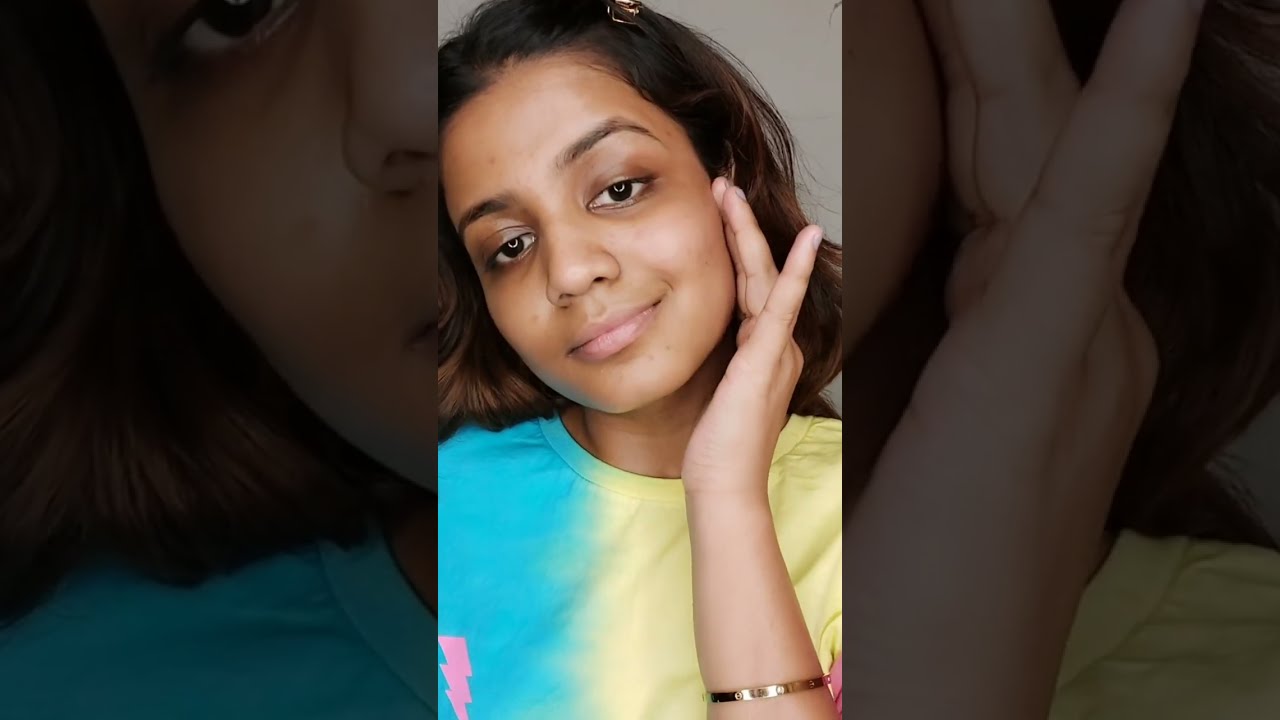The image depicts a young girl, possibly of Indian or Middle Eastern descent, with a caramel skin complexion and dark brown hair that reaches at least shoulder-length. Her hair is partially pulled back with a small barrette. She is centered in the image, which appears to be a close-up, horizontal rectangular selfie. She has large, expressive brown eyes that make direct contact with the camera, and her head is tilted slightly to her right, presenting a slight smirk. Her left hand, adorned with a gold bangle, gently touches her left cheek. She is wearing a vibrant tie-dye t-shirt with blue on the left side and yellow on the right, accented with hints of pink. The background is faded, keeping the focus solely on her. There is a natural, candid feel to the photograph, as if it was taken impulsively by herself or a close acquaintance.